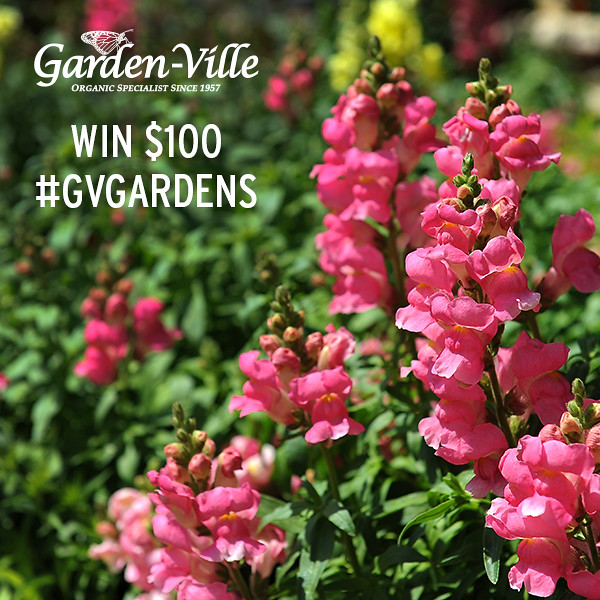The photograph captures a vibrant scene of pink peonies in full bloom, with lush green stems and leaves beneath them. The focal flowers form a spiraling tower-like structure, creating a striking contrast against the blurred background of similar pink flowers and a few distant yellow blooms. The sunlight from the upper left accentuates the vivid colors and natural beauty of the setting. In the upper left corner, the text "Gardenville" is prominently displayed in white font, with a delicate white outline of a butterfly perched on the "D." Below this, the text reads "Organic Specialist since 1957," followed by a promotion that states, "Win $100" and the hashtag "GV Gardens," all in white text.